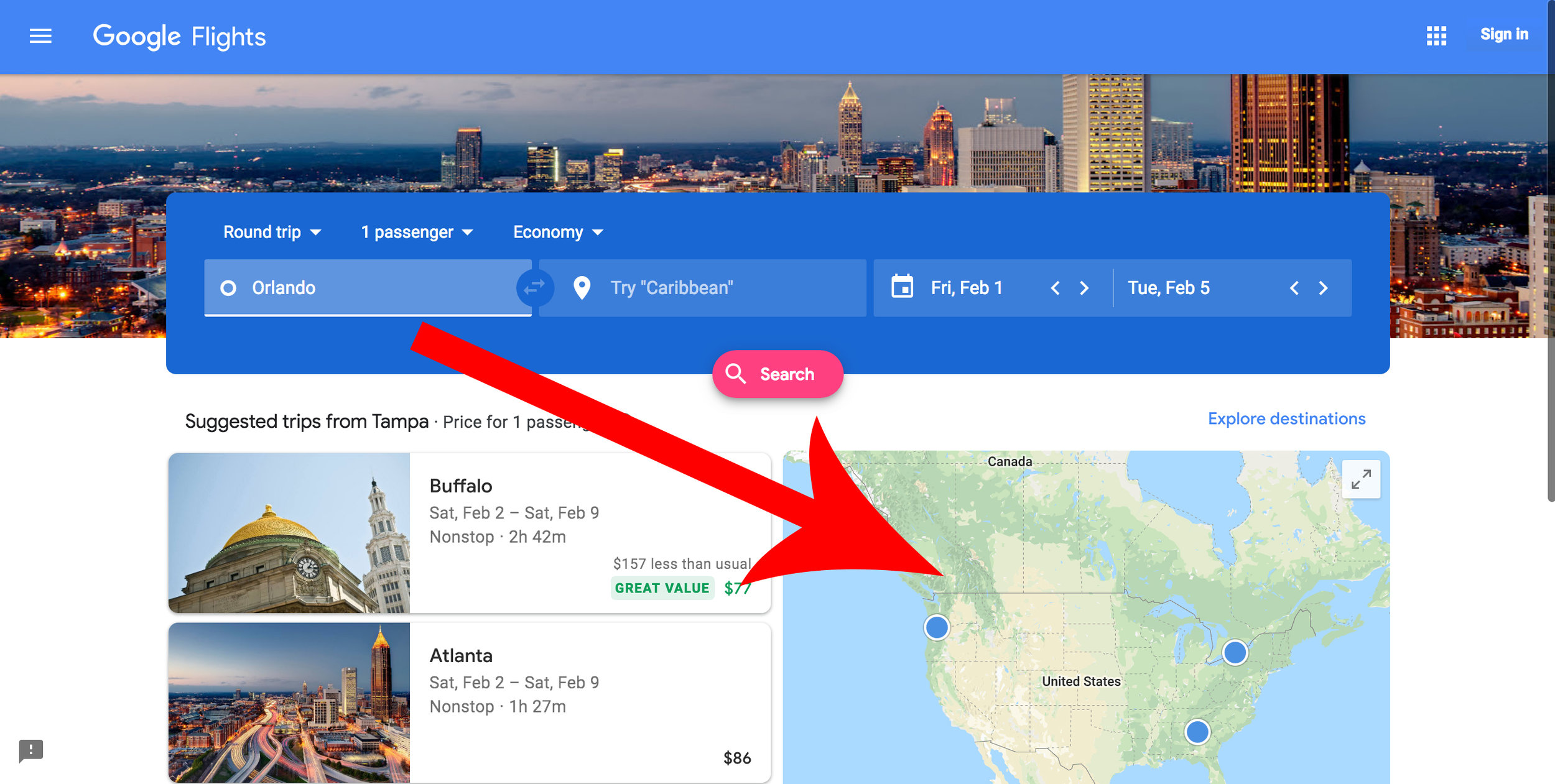The image depicts a nighttime cityscape with dark skies above towering skyscrapers, some of which have illuminated windows. In the foreground, there is a prominent blue rectangle displaying travel details: "Roundtrip, One Passenger, Economy," followed by the departure city, "Orlando," and the destination, "Tri-Caribbean." The travel dates shown are "Friday, February 1st" and "Tuesday, February 5th." 

Additionally, a color-coded wall features various annotated travel deals. A red and pink section highlights a red arrow pointing to the United States. Within this section, a deal for "Tampa" is detailed, priced for one passenger. Another deal for "Buffalo" lists specific dates: "Saturday, February 2nd to Saturday, February 9th," with a non-stop flight duration of "2 hours, 42 minutes," and a cost of "$157," noted as "less than usual, great value."

A different travel option for "Atlanta, Georgia" covers the same period, "Saturday, February 2nd to Saturday, February 9th," featuring a non-stop flight lasting "1 hour, 27 minutes," priced at "$86."

The bottom right of the image shows a global map segment, with Canada at the top and the United States below. Key locations are circled, indicating specific points of interest or travel routes.